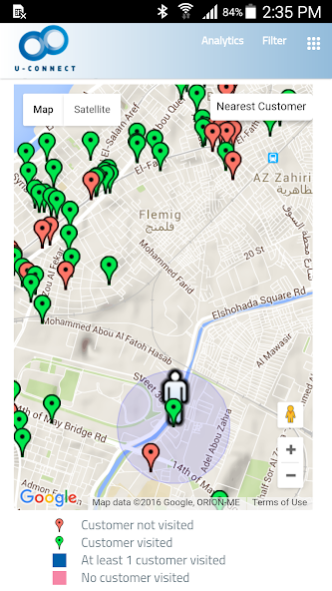The screenshot showcases the user interface of the UConnect mobile application, specifically focusing on the map view that provides detailed information about customer visits. At the top of the screen, the UConnect logo is prominently displayed alongside options for analytics and filters. The status bar shows the current time as 2:35 p.m., along with standard icons for battery life, Wi-Fi, and signal strength.

Dominating the screen is a detailed map, centered around the location labeled "Fleming," highlighting streets and landmarks. Numerous color-coded markers are dispersed across the map, each representing a different customer visit status: green markers indicate customers who have been visited, red markers signify customers who have not been visited, blue markers represent locations where at least one customer has been visited, and gray markers denote areas with no customer visits.

In the top left corner of the map view, there are buttons for toggling between map and satellite views, as well as a "Nearest Customer" button designed to find the closest customer location. At the bottom left, a legend clearly explains the color codes used for the markers, enhancing user comprehension. The bottom right corner features standard map controls, including zoom in and zoom out buttons, and a current location button for easy navigation.

This user-friendly interface efficiently combines visual representation and functional controls to provide a comprehensive overview of customer visit statuses, thus improving usability and productivity for the users.